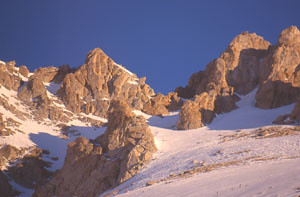The photograph captures a stunning mountain range with jagged peaks that rise above the snow, set against a vivid, cloudless blue sky. The image, which is horizontally oriented and approximately one and a half to two times as wide as it is tall, showcases a dynamic landscape where reddish-brown and grey rocky outcrops intermingle with patches of white snow. The snow cover varies in thickness, becoming more pronounced closer to the foreground and nearly absent at the mountain tops. Yellow streaks mar the rocky slopes, adding to the rugged beauty of the scene. The photo's bottom left corner reveals a valley, forming a bowl shape where the cliffs descend. Dark shadows cast to the left suggest the sun is positioned to the right, enhancing the texture and depth of the rocky and snowy surfaces.